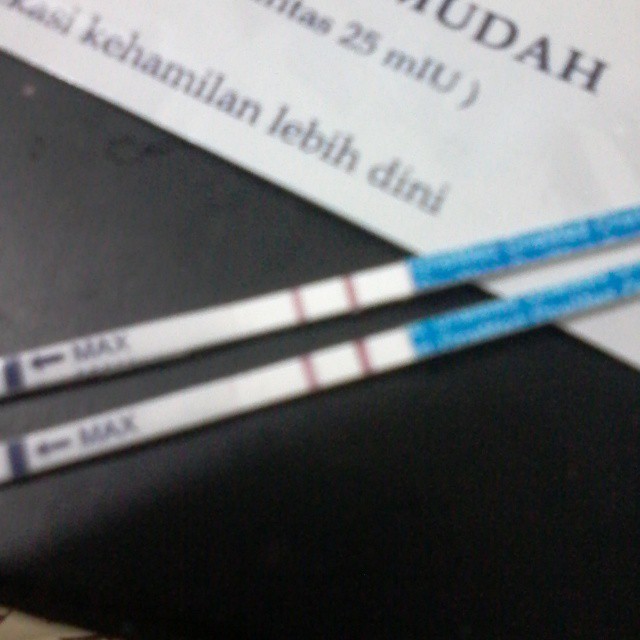This slightly blurry photograph features a predominantly black background with a small section of white visible in the bottom left corner. At the top of the image, there's a white piece of paper adorned with black text. The visible text reads "UDAH" at the top, followed by "LLAS 25 MIU" in the middle, and "KEHAM ILAN LEBIH DINI" at the bottom. Additionally, two objects resembling straws occupy part of the frame. These objects have a distinctive pattern, starting with blue sections featuring small lines at the bottom, followed by alternating sections of white and purple lines. The tip of each straw-like object is marked with the word "MAX" beside a black arrow, and the ends are highlighted in black.